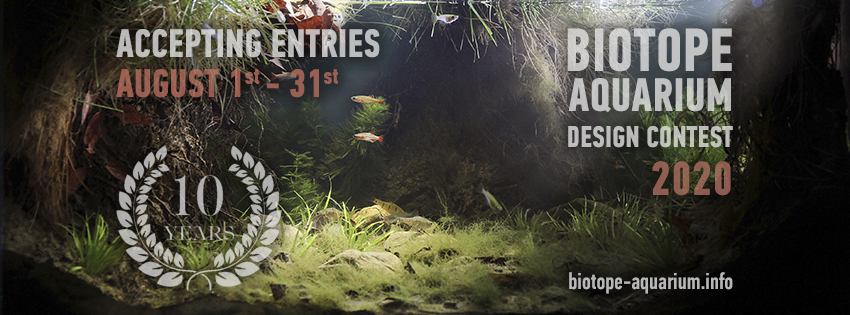The image is a poster in a horizontal rectangle format designed for an event. The scene depicted appears to be underwater, with the dark areas on the left and right sides and a brighter section in the middle showcasing green foliage, likely representing underwater plant life. The bottom of the image is lit up with grass or seaweed, and additional plants are scattered throughout the scene. There are three notable fish: two in the middle with a red and white design, possibly koi fish, swimming to the left, and a white fish, which resembles a shark, near the top middle. 

Overlaying the image, in the top left corner, are the words "ACCEPTING ENTRIES" in white capital letters, followed by "August 1st to 31st" in orange letters. At the bottom center, there is a white wreath encircling the text "10 YEARS." On the right side of the poster, the text "BIOTOPE AQUARIUM DESIGN CONTEST" is prominently displayed in capital white letters, with "2020" in orange below it. Finally, the website "biotope-aquarium.info" is located at the bottom right of the poster.